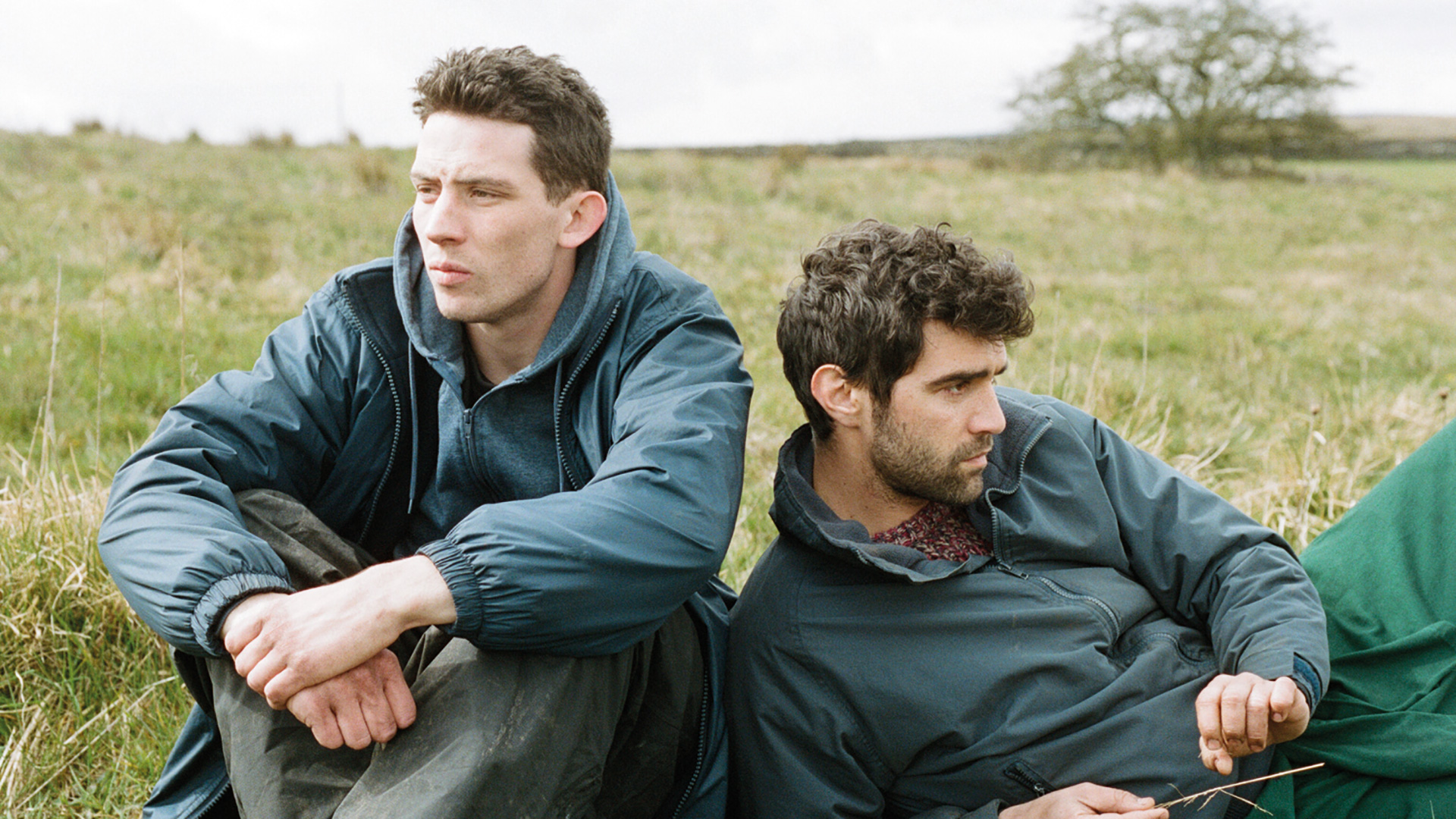In this photograph, two men are seen sitting in a field with a sparse, blurry tree in the far right background and a hill behind it. The grass is a mix of brown and green, under a dreary sky that isn't quite gray or blue. The man on the left, positioned just left of the centerline, has short, brown hair and a clean-shaven face. He is wearing a bluish nylon jacket with elastic cuffs over a zip-up hoodie, paired with grey slacks, and is sitting with his legs crossed, knees up, and arms resting on his knees, looking off into the distance. Beside him, the second man, also with brown hair that is somewhat curly, is reclined on his left forearm and elbow. He dons a similar blue windbreaker over a knitted sweater and green pants. He has a scruffy beard, mustache, and sideburns, and his shoulder is nearly touching the first man's hip. The composition suggests a quiet, contemplative moment shared between the two men amidst a subtly colored landscape.